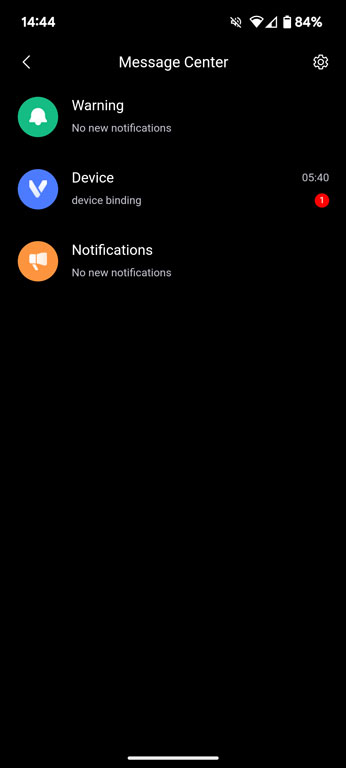The image is a screenshot from a mobile phone showing the interface of a notification center. At the very top of the screen, the time "14:44" is displayed, along with several icons, and the battery is at 84% charge. An arrow pointing to the left next to the label "Message Center" is also visible. On the far top right, there is a settings icon.

Below this, a notification section is visible. It begins with a white bell icon inside a green circle that indicates "Warning: no new notifications." Next to this, there is a depiction of a device folding, resembling the letter "V," within a blue circle. This section is labeled "Device" with a sub-label "Device Binding." Next to it, the number "0540" is displayed, accompanied by a red circle with the number "1" inside it, suggesting an unread item.

Further down, there is an orange circle containing a white emblem, labeled "Notifications." Below this, it reads "No new notifications."